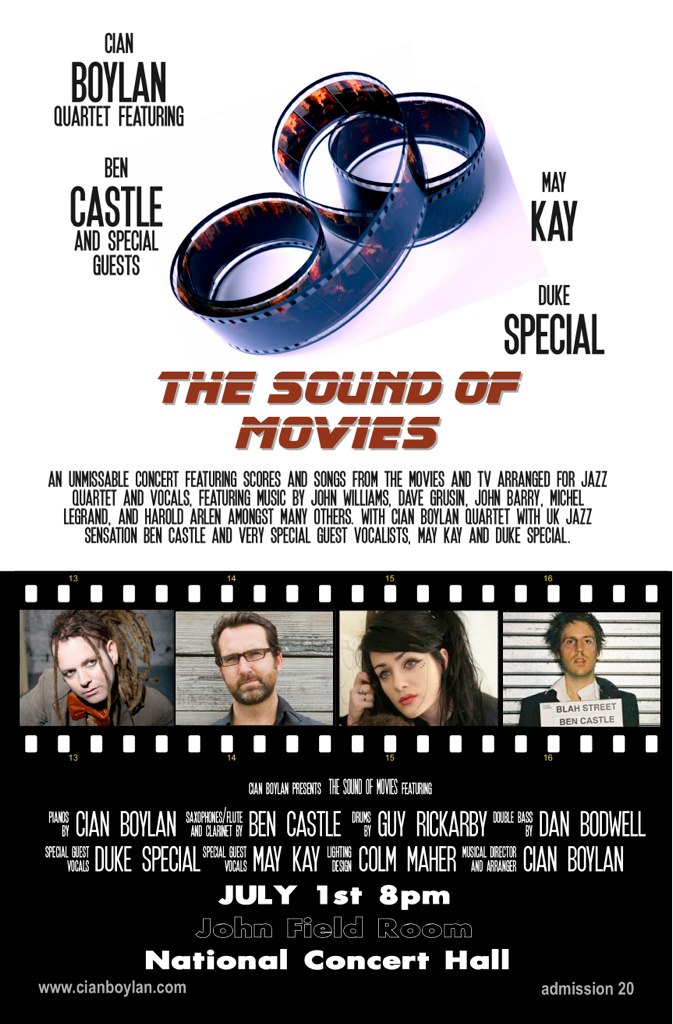This vertically formatted advertisement features a starkly contrasting layout with the background alternating between solid white and black sections. At the top, there are the names "Cian Boylan," with 'Boylan' more prominent, followed by "Quartet Featuring Ben Castle," emphasizing 'Castle'. Below, "And Special Guests" is stated, accompanying a central image of a coiled film reel, tinted blue, suggestive of embedded pictures.

Adjacent to the reel on the right are the names "May K," with 'K' larger, and "Duke Special," also highlighting 'Special.' Centrally, in bold red uppercase letters, the header reads "THE SOUND OF MOVIES," partitioned by a horizontal line. Beneath, there's a descriptive paragraph about the Cian Boylan Quartet.

The lower section, designed to mimic film strip aesthetics, showcases four headshots: a young woman in a gray shirt, a bearded man with glasses, another woman with long hair, and a disheveled man noted as 'Dean Castle,' all appearing serious. Concluding the design, detailed information about the event is listed in a black rectangle, formatted like movie credits, featuring the date "July 1st, 8 p.m." and location "John Field Room, National Concert Hall," with additional details in the bottom corners, presumably the website and admission cost.